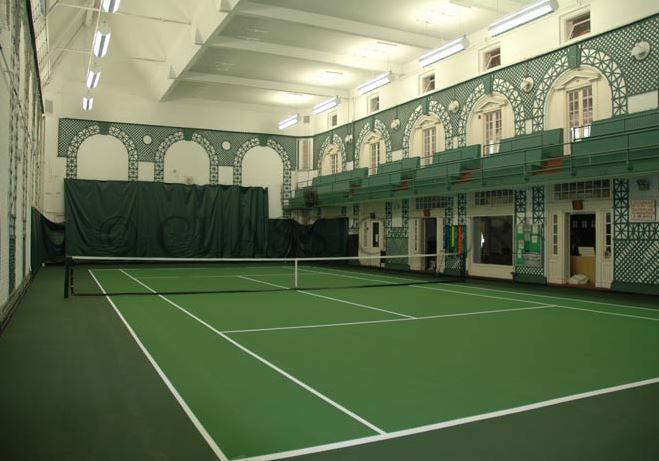This image depicts a large, indoor tennis court set within a fairly old-fashioned and ornate building. The court itself is bright green with white regulation lines and a net strung across its center. Surrounding the court are tall white walls adorned with a green design of painted arches, which extend around the interior. Alongside the long wall of the tennis court, towards the back, stands a tall green barrier seemingly designed to prevent tennis balls from escaping. Elevated high on the right side, there is balcony seating with a couple of rows of green benches, accessible via doorways that feature intricate stenciling, ornamental covers, and off-white shutters. Overhead, the white ceiling is supported by various beams and illuminated by fluorescent lighting, adding to the structure's grandeur. The space is devoid of players, allowing a clear view of its architectural and functional details.